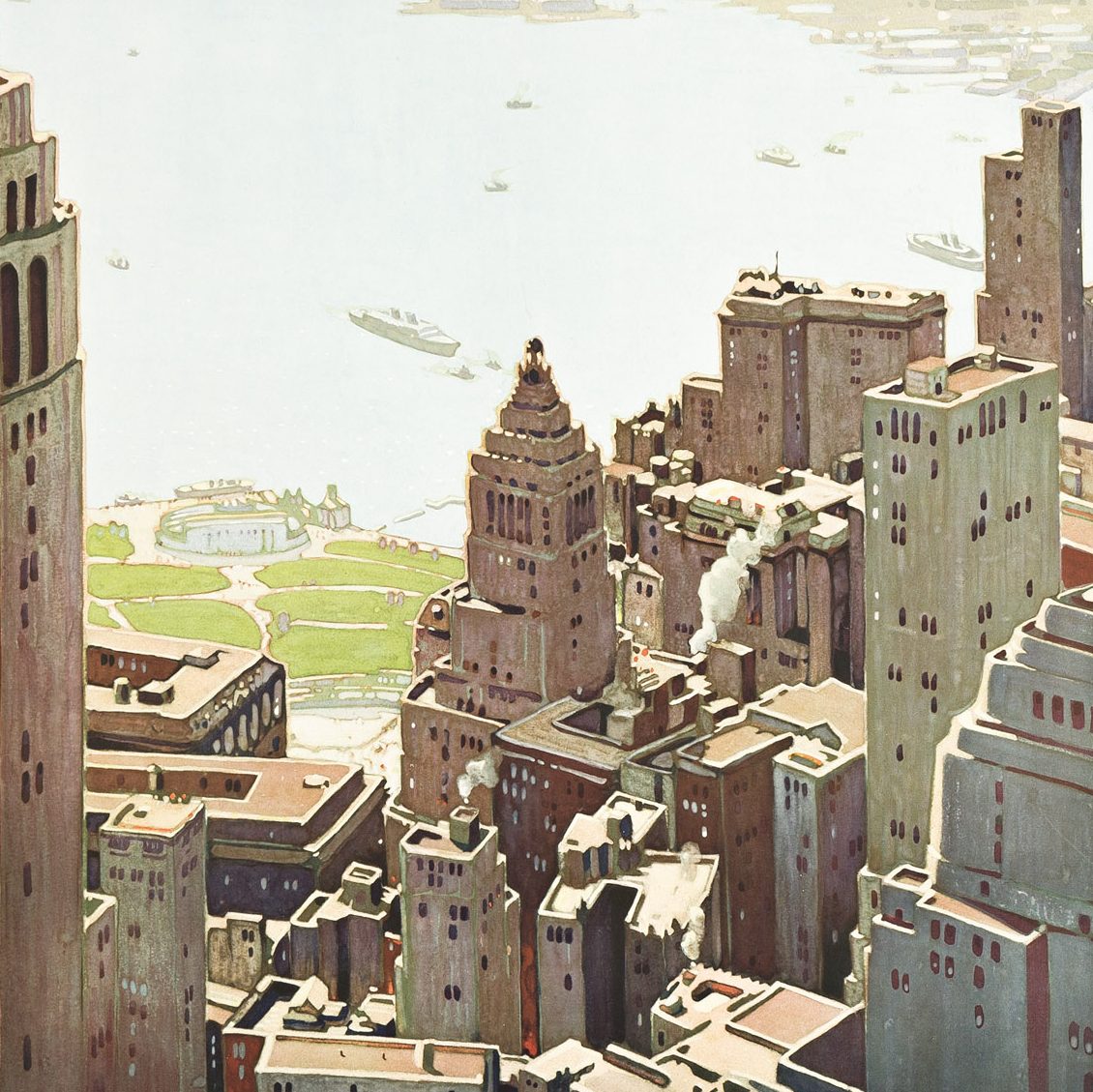This image appears to be a detailed painting of an old city with numerous tall, closely-packed buildings in shades of brown and light brown, exuding an historical ambiance. In the foreground, among the dense cluster of high-rises, smoke billows from one of the chimneys, hinting at industrial activity. Present in one part of the city, perhaps on the left-hand side, there's a patch of greenery, possibly a park. The scene extends to the backdrop where a muted, grayish-cream body of water, dotted with small boats, stretches out into the horizon. Some boats are more distant, adding depth to the scene. The artwork is characterized by its subdued and muted color palette, potentially indicating a watercolor technique, and lacks a frame or any identifying information about the artist or the depicted city.